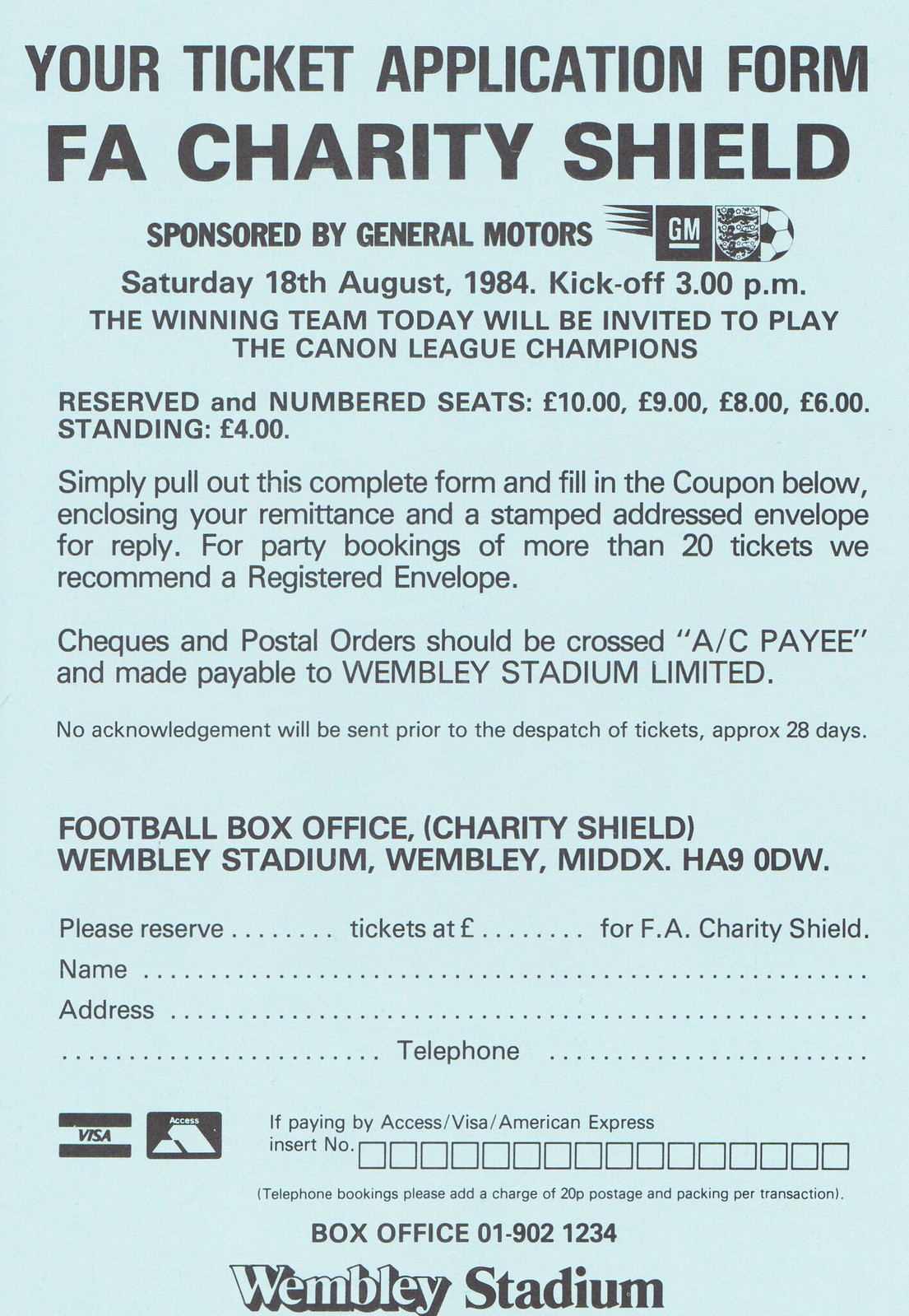The image depicts a light blue paper application form for event tickets, with black text detailing important information. At the top, it reads "Your Ticket Application Form" for the F.A. Charity Shield, sponsored by General Motors, accompanied by a logo featuring a soccer ball. Below, it states the event date, "Saturday, 18th August 1984," with a kickoff time of 3 PM, and mentions that the winning team will be invited to play in the Canon League Championships.

The form lists ticket prices: reserved seats at £10, £9, £8, and £6, with standing tickets at £4. It instructs applicants to complete the form and submit it along with payment, enclosing a stamped addressed envelope for a reply. For orders exceeding 20 tickets, a registered envelope is recommended. Checks and postal orders are to be crossed A/C and made payable to Wembley Stadium Ltd. No prior acknowledgment will be sent before ticket dispatch, expected approximately 28 days before the event.

The bottom section of the form includes fields for personal details: name, address, telephone number, and ticket quantity requests. It mentions additional charges for telephone bookings and provides contact information, including the Football Box Office at Wembley Stadium, with the address "Wembley Stadium, Wembley Medics, HA90DW," and a contact number: 01-902-1234.